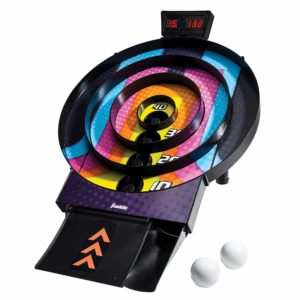In this image, we see a vibrant, pinball-style toss game against a pure white background, typical of e-commerce website presentations. The center of the game features a colorful circular target area with concentric rings marked with varying point values: the innermost ring scores 40 points, followed by rings scoring 30, 20, and 10 points. The target area is adorned in bright hues of blue, pink, yellow, and orange. A red digital scoreboard displaying the game's score is prominently positioned at the top. Below the target area, a black ramp with three orange arrows directs the balls towards their respective point zones. Two white balls, resembling ping pong balls, are placed to the right of the game, ready for play. This setup, reminiscent of the kind of game found in an arcade, invites players to roll the balls into the target rings to accumulate points.